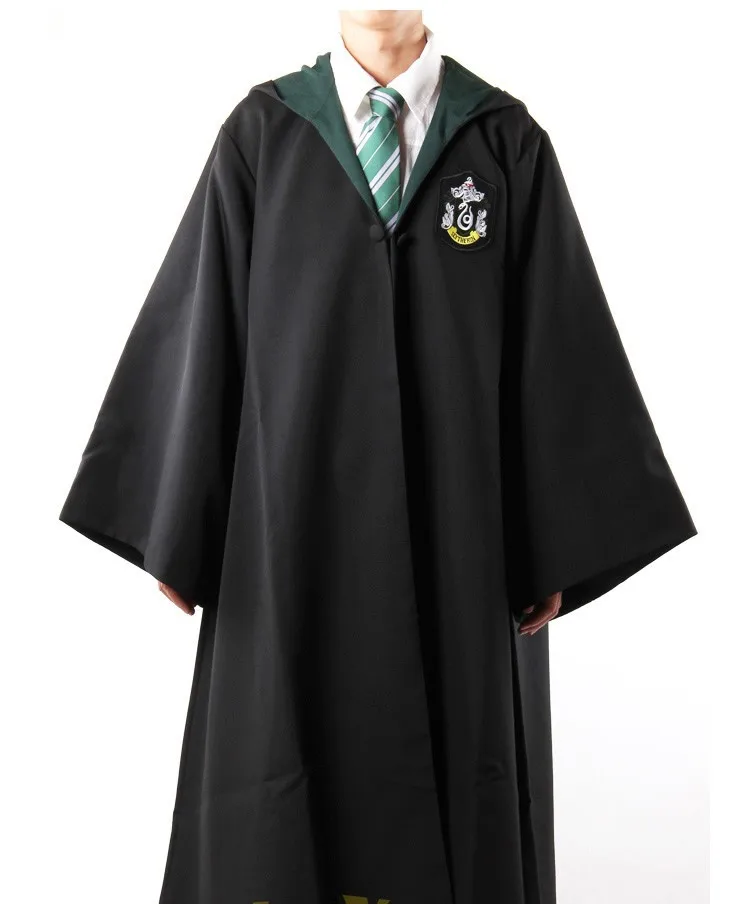In this image, a person is depicted from the neck down, wearing a distinctive black graduation gown with an attached hood. Only the lower part of their face, specifically their chin and neck, is visible; no other facial features are shown. The individual's hands are slightly poking out from the oversized, baggy sleeves. Underneath the gown, they are dressed in a neatly collared white shirt paired with a green and white striped tie. 

The background is plain white, emphasizing the details of the attire. On the left chest area of the gown, which appears on the right side of the image due to the person's orientation, there is an emblem featuring a white top section and a yellow curved bottom with a swirl in the center, although the exact design is not clear. The person has a lighter complexion, conveying an organized and clean appearance.